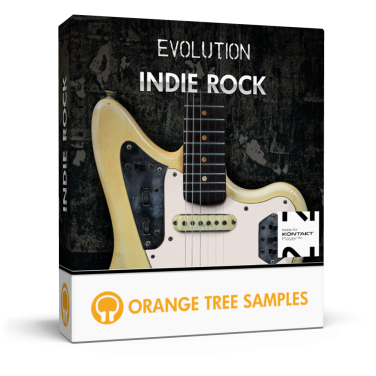The image depicts a square box set titled "Evolution Indie Rock," prominently featuring a close-up photograph of the top part of an electric guitar. The guitar has a black neck and a dark ivory-colored body with a black inlay on the left side and the rest of the body in white. The fretboard of the guitar is a lighter ivory color. The background of the image is a montage of darker photographs, creating a layered effect behind the guitar. Along the spine, the title "Indie Rock" is also displayed. The bottom section of the box is white, featuring an orange logo with a pair of white headphones inside, and the text "Orange Tree Samples" next to it. The box appears to be several inches thick, suggesting it may contain multiple items, perhaps a collection of music.